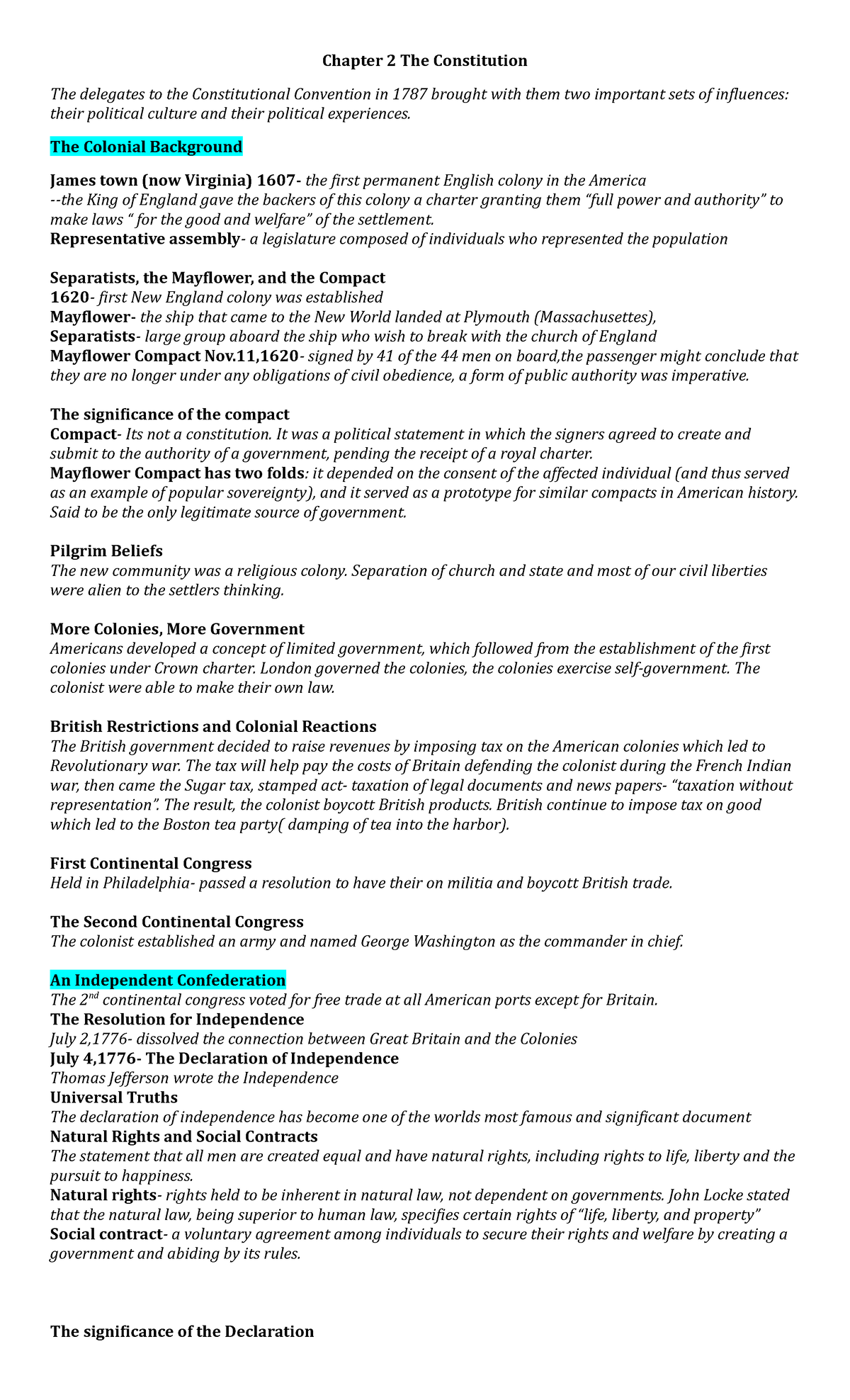This image captures a smartphone displaying a page from an e-book, specifically opened to Chapter 2, titled "The Constitution." The page delves into the colonial history of the United States, beginning with the founding of Jamestown in 1607, noted as the first permanent English colony in America, located in present-day Virginia. The text highlights key historical elements such as the Separatists, the Mayflower, and its Compact, emphasizing the significance of the Compact in shaping early American governance. Subsections discuss Pilgrim beliefs, the establishment of more colonies and governments, British restrictions, and colonial reactions.

Highlighted sections draw attention to "Colonial Background" at the top and "An Independent Confederation" towards the bottom of the page. The narrative transitions through key periods, mentioning the First Continental Congress, the Second Continental Congress, and moves towards the development of an independent confederation.

A specific portion of the page elaborates on the representative assembly, describing it as a legislative body composed of individuals who represented the population. The text points out that the backers of the Jamestown colony received a charter from the King of England, granting them full power and authority to enact laws for the welfare of the settlement. The section concludes with the significance of the Declaration, rounding out an in-depth exploration of early American constitutional development.